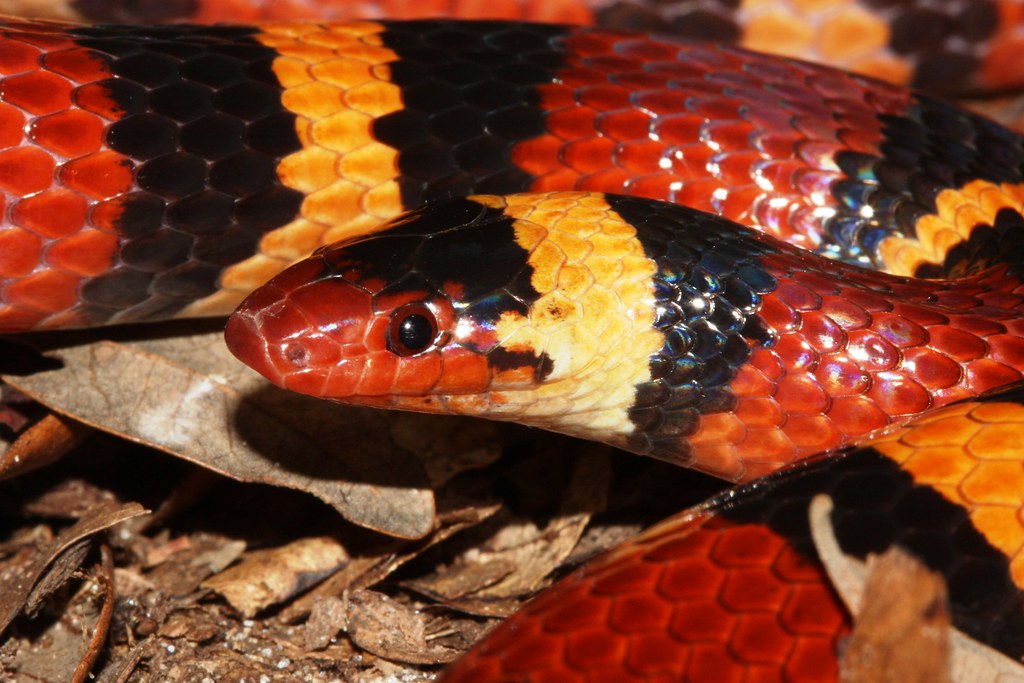The detailed close-up photograph captures a calm, coiled snake set against a natural backdrop of brown leaves and soil, evoking a wild animal setting. The snake's intricate pattern of alternating wide red, and narrower black and yellow bands runs the length of its glossy, leathery body. The head, which is slightly elevated, is positioned centrally in the vertical frame, revealing its red eyes and closed mouth. The detailed texture of the snake's skin showcases hexagon-shaped scales, enhancing its glossy appearance. The overall color sequence of dark orange, black, and dark yellow repeats rhythmically along the body, emphasizing the snake's striking and vibrant color palette. The atmosphere suggests an autumn setting, with the ground's earthy tones complementing the snake's vivid hues. The photograph, despite the snake’s potential danger, highlights the serpent’s natural beauty and intricate details.